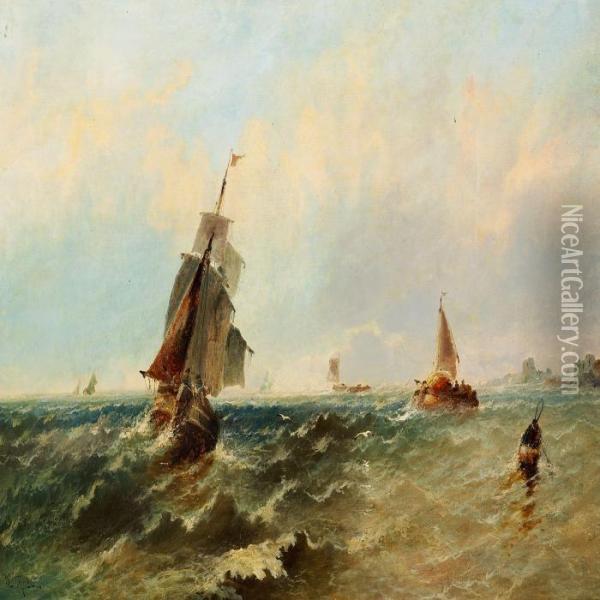The painting depicts a dramatic seascape from presumably the 17th or 18th century, characterized by multiple large sailboats navigating a tumultuous ocean. The artist has captured the rough seas using a palette of dark blue, light blue, white, and hints of brown and green, evoking a sense of danger as the ships struggle against the choppy waves. The ships, equipped with old, ragged sails in shades of brownish and white and red, are being tossed about by the stormy waters. To the right side of the painting, a faint watermark reads "NiceArtGallery.com," marking its provenance. The sky above is a mix of cloudy hues, from pale blue to dark blue with touches of gold, suggesting a storm or the remnants of one. In the background, faint silhouettes of city buildings imply nearby land, contributing to a scene where the vessels might be approaching a harbor. The overall composition masterfully conveys the movement and intensity of the sea, creating a vivid and historical maritime atmosphere.